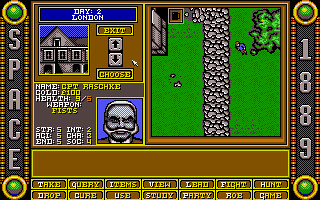The screenshot captures a vintage-themed video game interface titled "Space 1889." The screen is bordered by labels on either side: "space" vertically aligned on the left, and "1889" similarly on the right. Each corner is highlighted by a green dot encircled in yellow, adding a unique, decorative touch.

The central part of the screenshot displays the main walkthrough scene of the game. On the left side, a blue label indicates the current setting with the text "Day Two, London." Below this label, a small, square picture of a man's face is shown, accompanied by his name, gold count, health status, and current weapon. Surrounding this, various character stats provide detailed information about the player's progress and condition.

Adjacent to the main gameplay area, a house within a square is visible, suggesting a designated location or important objective point. Below, the word "Exit" likely functions as an interface element to leave or move to another screen. Directly above "Exit," two vertically stacked buttons labeled "Up" and "Down" appear, presumably for navigation.

At the bottom of the screen, an array of action buttons provides player commands: "Take," "Drop," "Query," "Cure," "Items," and "Use." These commands offer a range of interactive options for engaging with the game environment and managing inventory.

Overall, the intricate details and period-specific design of the interface draw players into the immersive world of "Space 1889," offering a nostalgic yet engaging gaming experience.